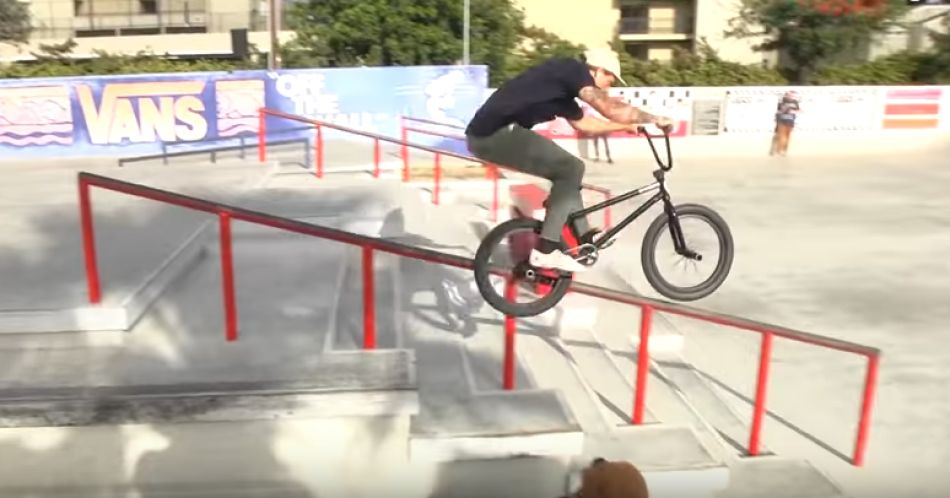In this photo, a daring young man is captured mid-air while performing a stunt on a black bicycle descending a flight of concrete steps. He is in a dynamic skatepark-like arena adorned with red, rusted rails that outline the steps. The skateboard park has a gritty urban feel, with walls surrounding the area and a concrete pit at the bottom of the stairs. An advertisement for Vans is visible in the background, adding to the skate culture vibe. 

The man, dressed in a dark blue t-shirt, gray pants, and white tennis shoes, sports distinctive tattoos on his arm and wears a white or tan baseball cap. His fearless stunt takes place under a clear sunny sky, enhancing the vibrant urban setting. In the background, there are some trees, several buildings, and a blurred figure standing near a wall, possibly watching the impressive display.